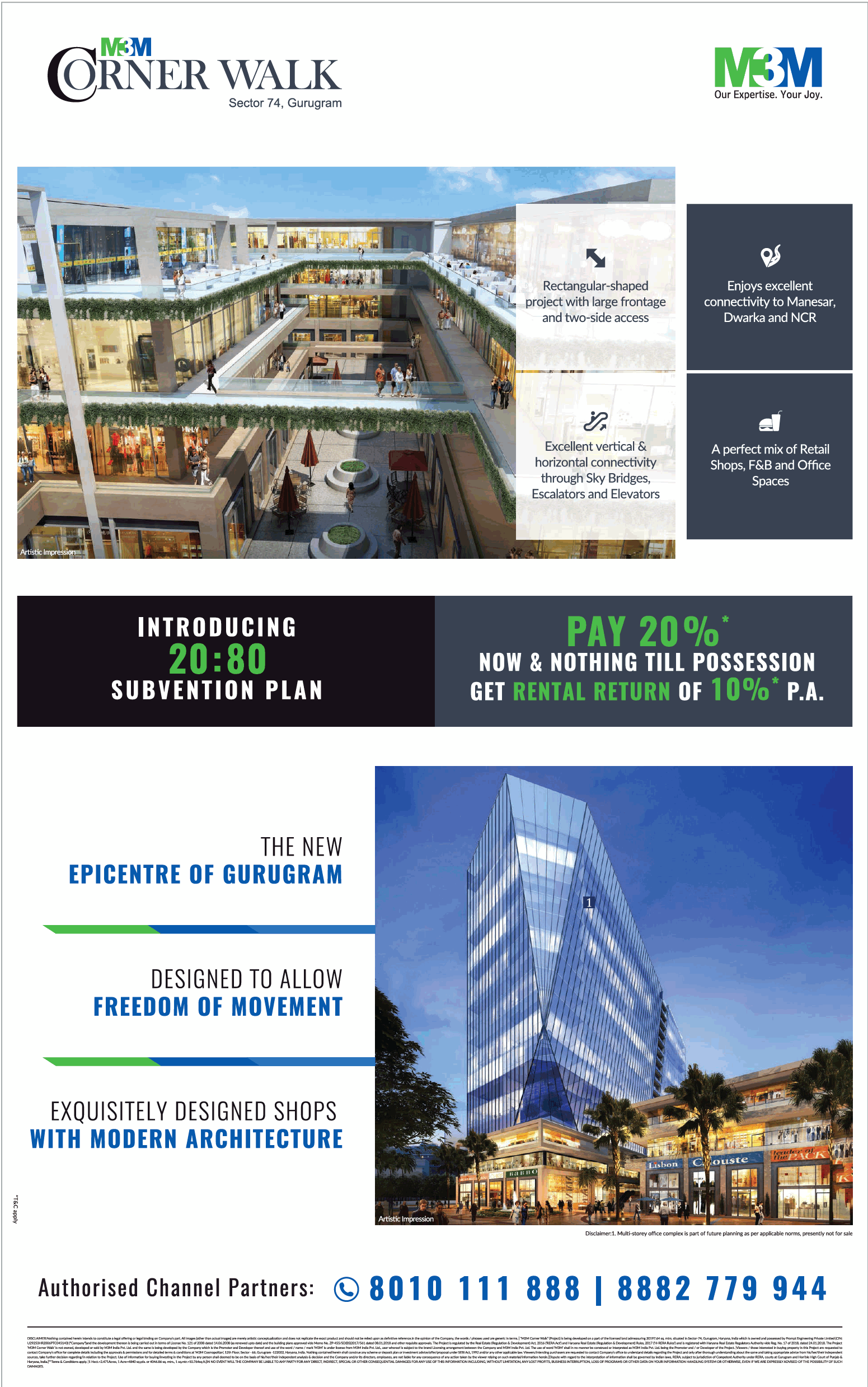The promotional image features a company advertisement with a sleek design on a clean white background. In the upper right-hand corner, there is a prominent M3M logo. The logo consists of a green "M", a white "3", and a blue "M". Just below the logo, the tagline "Our Expertise, Your Joy" is displayed.

In the upper left-hand corner, the same M3M logo is shown with additional text: "Corner Walk, Sector 74, Gurugram". The central area of the image showcases an artist’s rendering of a modern mall with multiple floors adorned with cascading green ivy from the walkways, adding a touch of nature to the contemporary setting. 

Text on the image describes the mall as a "rectangular-shaped project" boasting a large frontage and two-sided access. It highlights excellent vertical and horizontal connectivity through the use of sky bridges, escalators, and elevators. The mall also boasts excellent connectivity to Manesar, Dwarka, and the NCR region. 

The promotional message emphasizes a perfect mix of retail shops, food and beverage outlets, and office spaces within the development. Additionally, it introduces a "20 AV subvention plan", allowing buyers to pay 20% upfront with no further payments required until possession. A rental return of 10% is also promised. The caption finishes by describing the development as the "epicenter of Gurugram," designed for free movement and featuring exquisitely designed shops with modern architecture.

For further details, the image lists authorized channel partners with contact numbers: 8010-111-888 and 882-779-944.